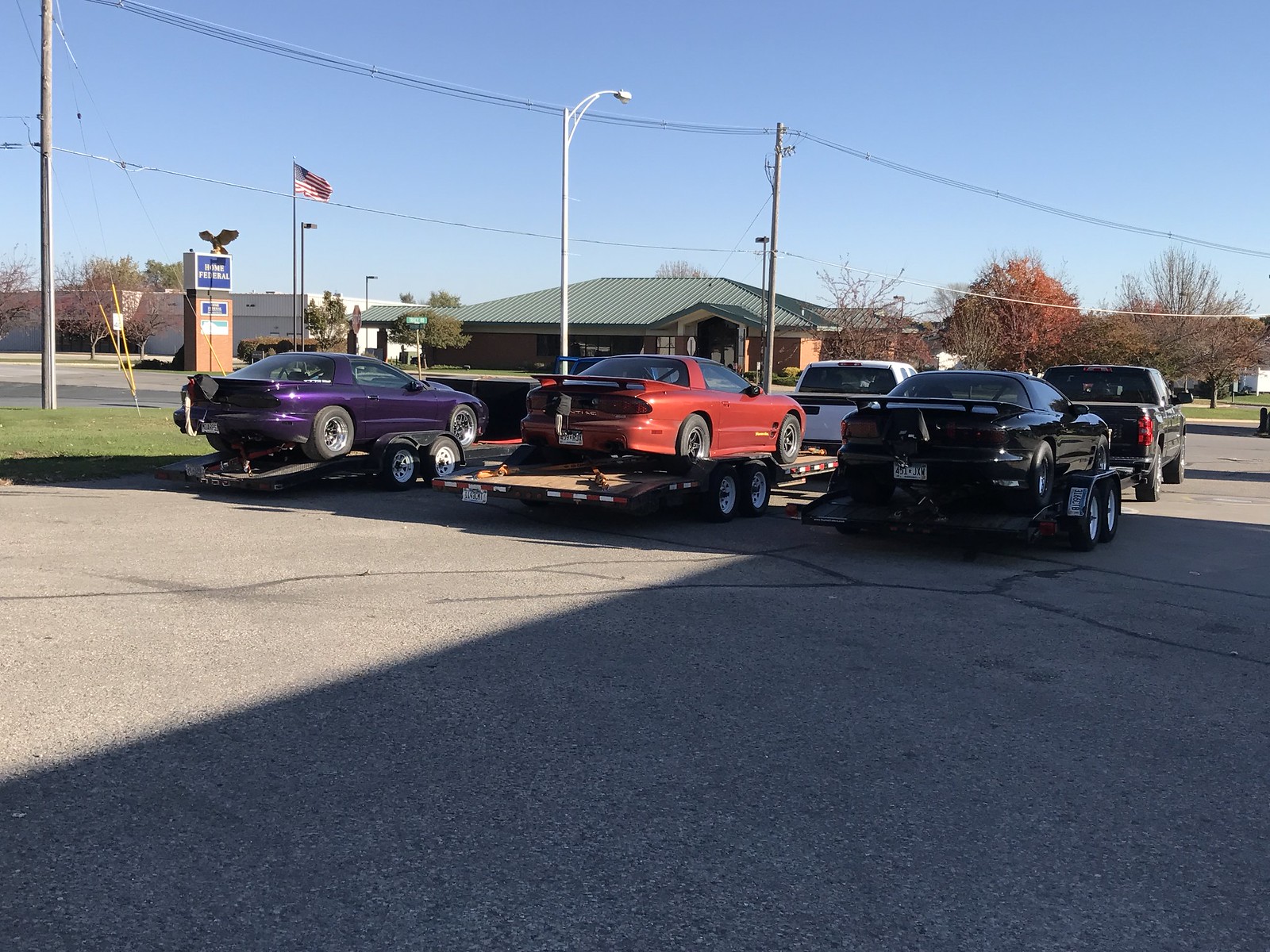In a sunny parking lot with patches of tar on the asphalt, three tandem axle trailers are lined up, each carrying a sports car. Shadows stretch out from the right side while the bright blue sky with few clouds occupies the upper quarter of the image. Across the street, a blend of buildings, including what looks like a financial center with a sign that mentions "Federal" and an eagle emblem, stands out. The bank-like building is also accompanied by an American flag, streetlights, and low deciduous trees. The focus returns to the vehicles: the trailer on the far left carries a blue car and is pulled by a barely visible blue pickup truck, the middle trailer carries a red car pulled by a white pickup truck, and the far right trailer holds a black car, being towed by a black pickup truck. In the far background, a large white building looks abandoned but remains in decent shape, adding to the scene's complexity and detail.